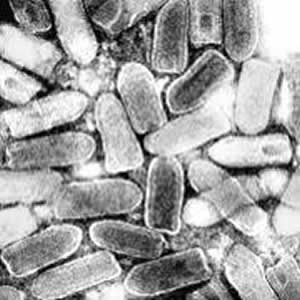The image displays a tightly-packed group of cylindrical, bullet-shaped objects, varying in shades from light gray to dark gray and some almost black. These objects have one flat end and one rounded end, resembling capsules or microorganisms typically seen under a microscope. The black-and-white image lacks a border and text, with all the items closely grouped together, leaving little space between each. In the upper right corner, a solid white area suggests a source of light. Some bullets have black spots, and they appear to be outlined in white, enhancing the contrast within the image. The overall appearance of the objects and their arrangement evoke the microscopic view of cells or bacteria.